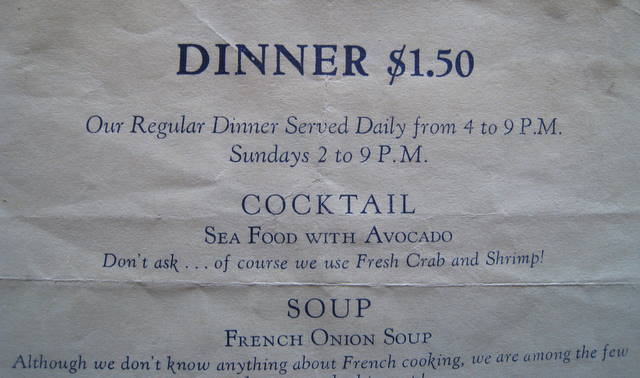Certainly! Here's the cleaned-up and detailed descriptive caption:

---

This image showcases a vintage restaurant advertisement or menu elegantly printed on whitish-gray paper with a clean layout and centered typography. 

At the top, in bold black all-capital letters, the central focus reads: **DINNER $1.50**. Below this, a clear description informs patrons: *"Our regular dinner served daily from 4 to 9 p.m. Sundays 2 to 9 p.m."*

As the eye moves down, the menu highlights key offerings in bold all-capital letters:

**COCKTAIL**  
**SEAFOOD WITH AVOCADO**

In a playful script font, it adds: *"Don't ask... of course we use fresh crab and shrimp!"* 

Further down the page, another bold heading reads:

**SOUP**  
**FRENCH ONION SOUP**

In the whimsical script font, it teases: *"Although we don't know anything about French cooking, we are among the few..."* (The rest of the sentence is cut off, leaving the reader intrigued.)

The entire layout is artfully designed, with ample margins on either side, ensuring a neat and engaging presentation. It emphasizes the affordability and daily availability of the dinner special, inviting diners to enjoy a meal until 9 p.m. each day.